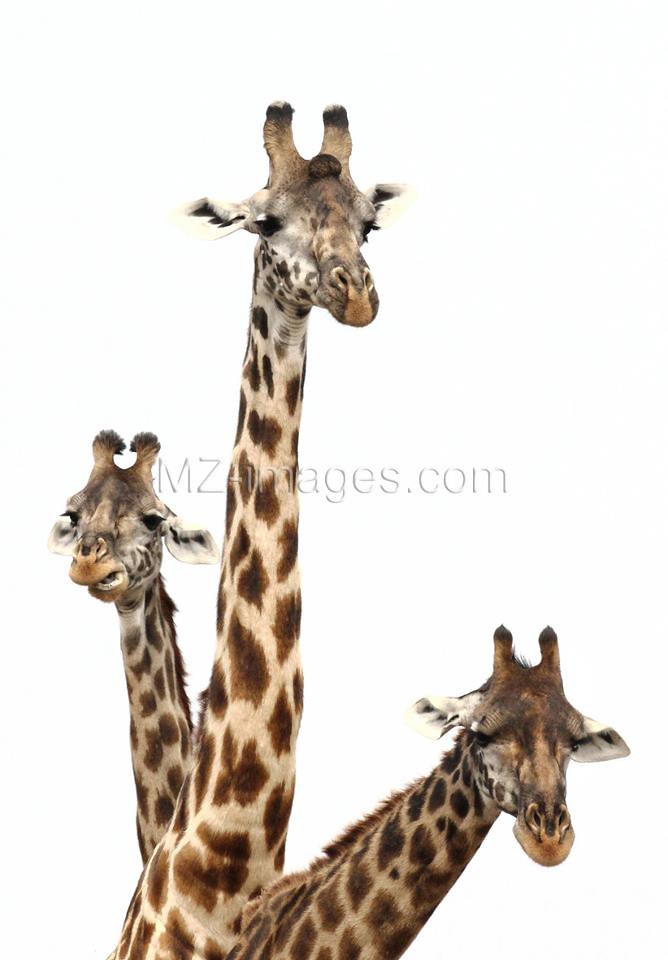This is a detailed color photograph of three giraffes, prominently displaying their necks and heads against a solid white background, likely achieved by background removal. The watermark "mz-images.com" is visible across the front center portion of the image. The giraffes, which vary in size, are all facing the camera, showcasing their characteristic features: flat faces, eyes positioned on the sides of their heads with long eyelashes, small horns (ossicones), and rounded mouths. Each giraffe exhibits the distinctive tan, reddish-brown color with patterned spots, although their bodies and legs are not visible, focusing the view from the base of their necks to the tops of their heads. One giraffe has its mouth open while the other two have their mouths closed.